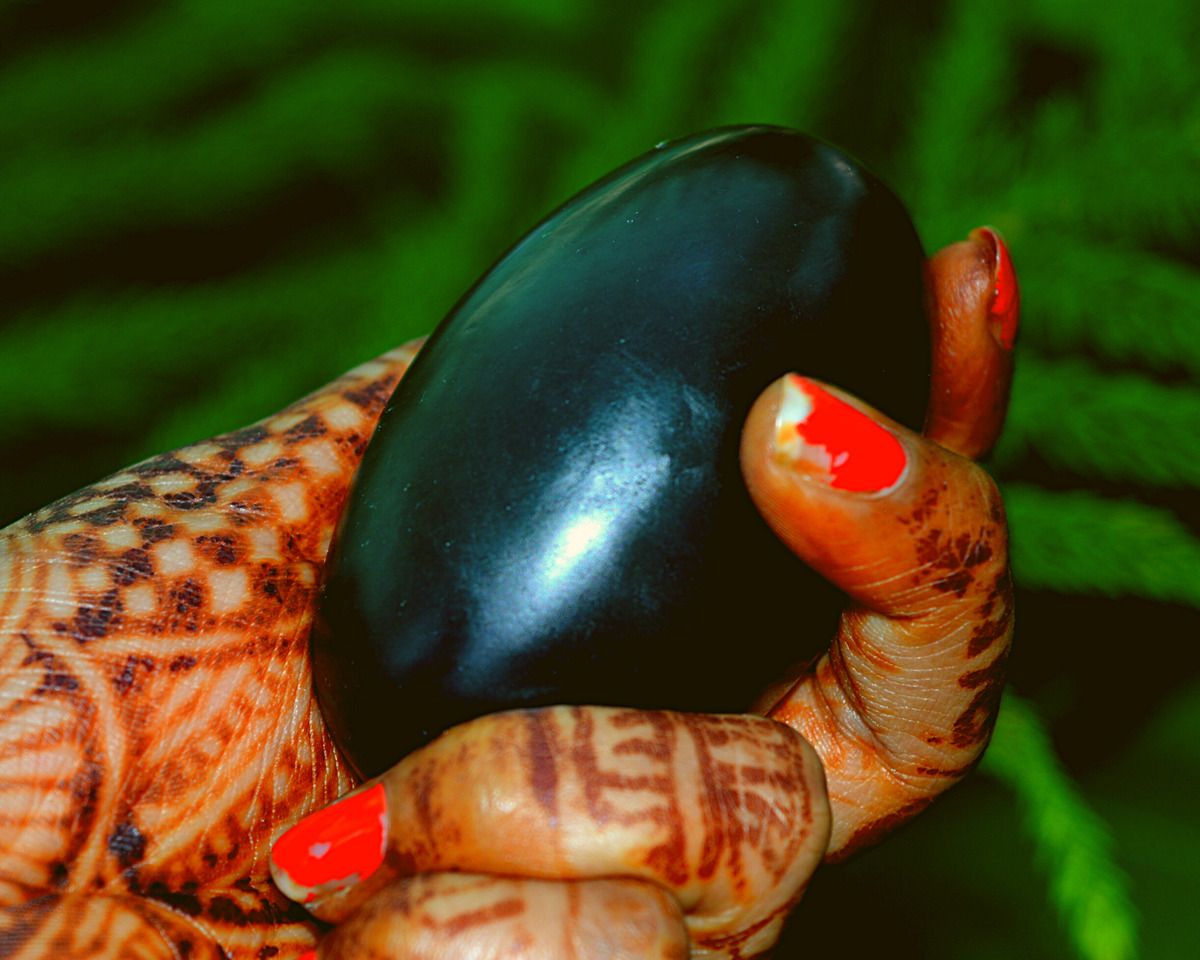In this captivating image, a woman's left hand, adorned with intricate henna tattoos displaying swirls, checker mark patterns, and zigzag designs, holds a smooth, shiny, oval-shaped black object, resembling a mango in size but with the glossy appearance of an eggplant. Her red nail polish is notably chipped, adding a touch of rugged character to her otherwise meticulously decorated hand. The background features an out-of-focus array of long green foliage, with some pine needles coming into sharper view on the right side of the frame, creating a natural yet blurred backdrop that enhances the intriguing presence of the mysterious black fruit-like object she holds.